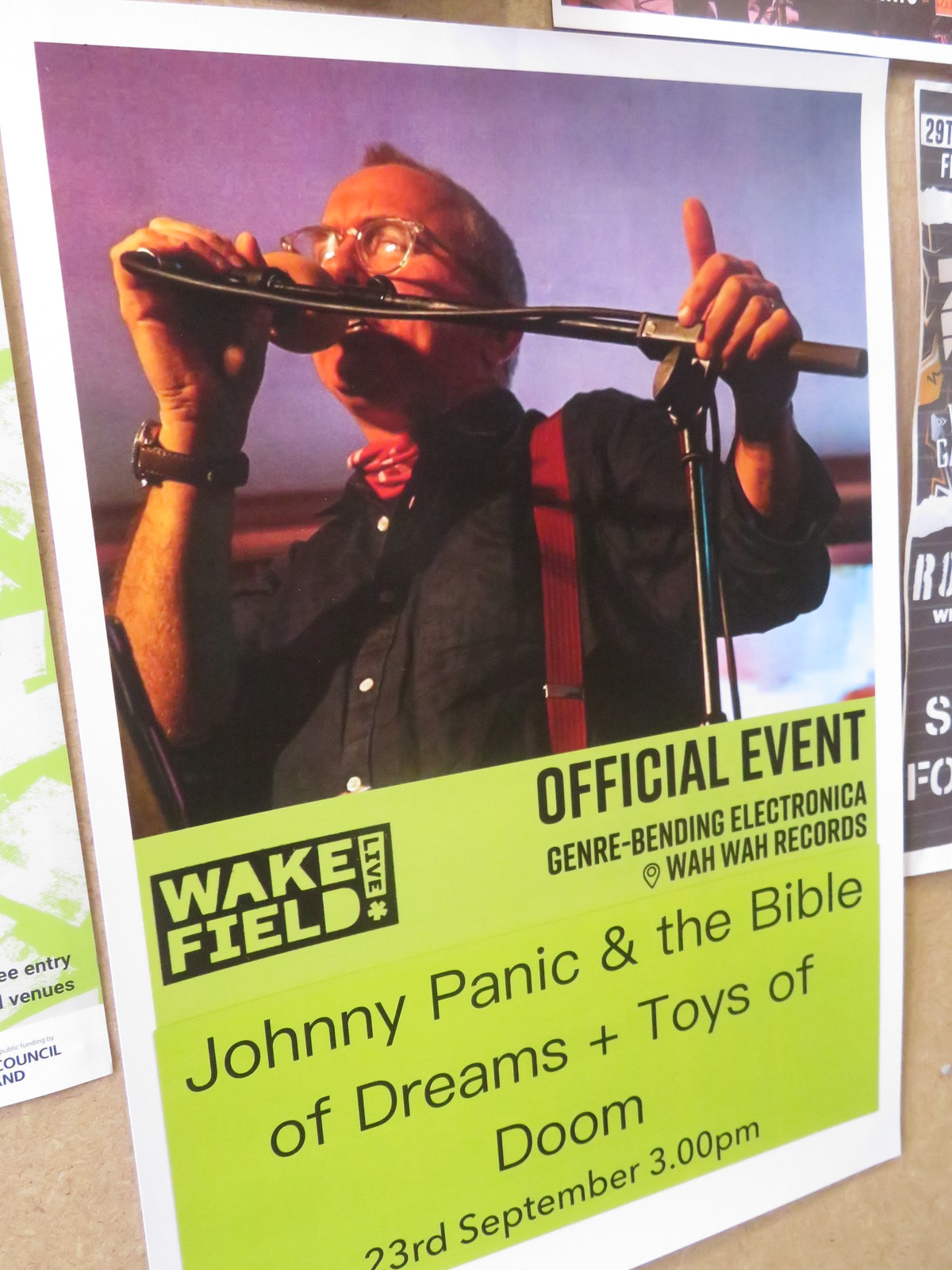The image is a vertically aligned, portrait-orientation photograph showcasing a large, color poster affixed to a tan-colored corkboard, with edges of other posters visible on the left and right sides. The featured poster is framed with a white border and split into two distinct halves. The top half is a close-up photograph of an older white man singing into a microphone on a stand. He has short gray hair, wire glasses, and a brown watch on his right wrist. The man wears a black button-down shirt with red suspenders, and the image is cut off just around his waist. The photograph is taken from a low angle, giving the impression that we are looking up at him. The backdrop of this top section is a purplish-blue color.

The bottom half of the poster has a lime green background with printed black text. It prominently features the phrases "Wakefield Live" and "Official Event" in bold letters, followed by "Genre-Bending Electronica" and "Wawa Records." The central text promotes performances by "Johnny Panic and the Bible of Dreams" and "Boys of Doom." The event's date and time, "23rd September 3 PM," are listed at the bottom. This descriptive and detailed poster effectively advertises a music event, merging visual and textual elements seamlessly.